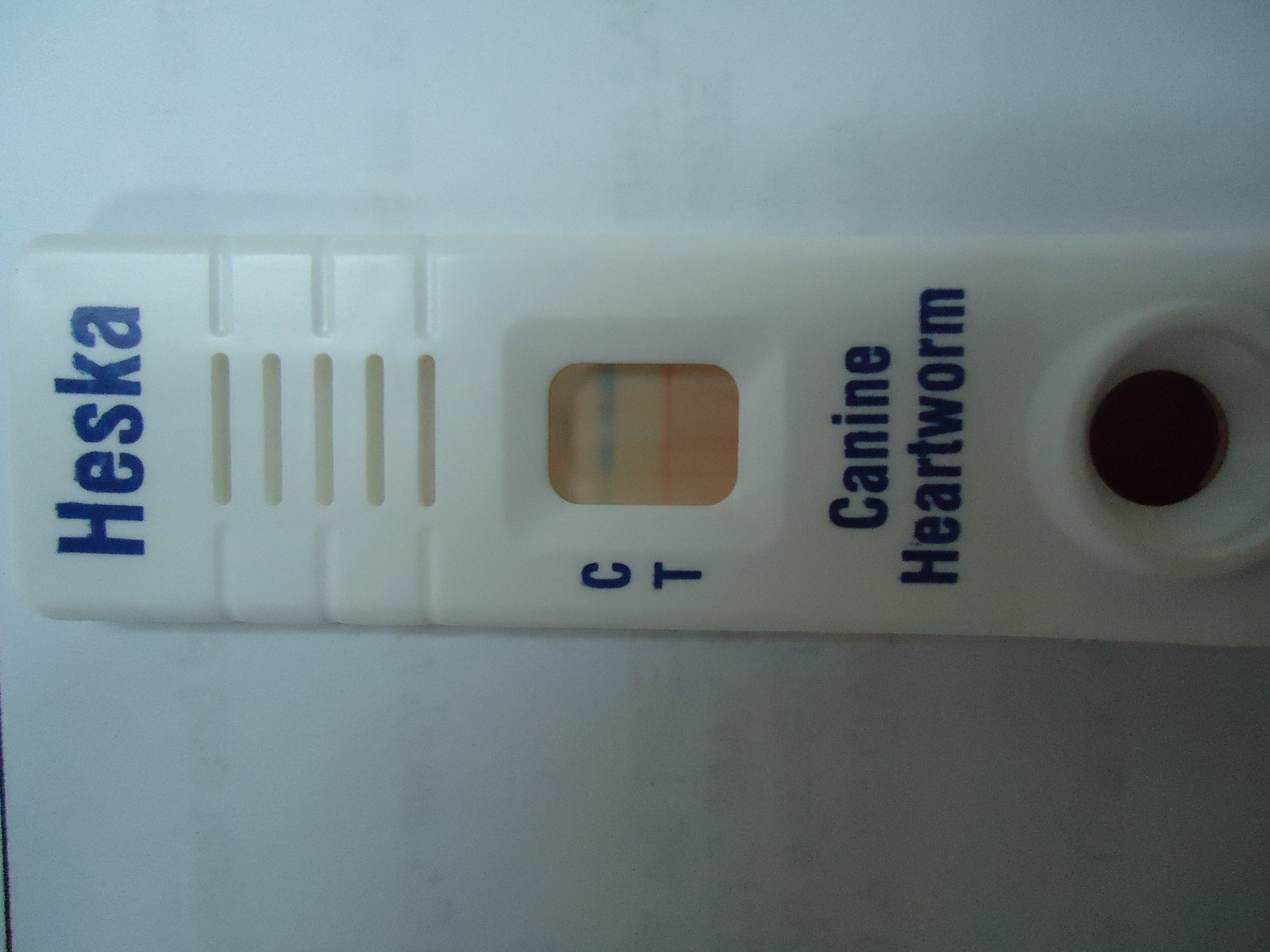In a room with white walls, a piece of specialized equipment is mounted in the center. The device, rectangular in shape, is predominantly white and features bold blue lettering at the top that spells "HESKA." Below the brand name, the equipment has five slender, vent-like openings arranged in a row, providing a distinct yet unassuming design feature. Additional vent markers are present on the sides, aligning with the first, third, and fifth openings.

A small display on the device stands out due to its bright orange background, on which the abbreviation "CNT" is prominently displayed. Within this display, a green line appears next to the 'C', and a pink line is adjacent to the 'T'. Below this display, the words "K-9 Heartworm" are clearly inscribed, indicating the device’s purpose as a diagnostic tool for detecting heartworms in dogs. Further down, a circular input area is visible, likely intended for sample collection—potentially saliva or another relevant substance used in the testing process.